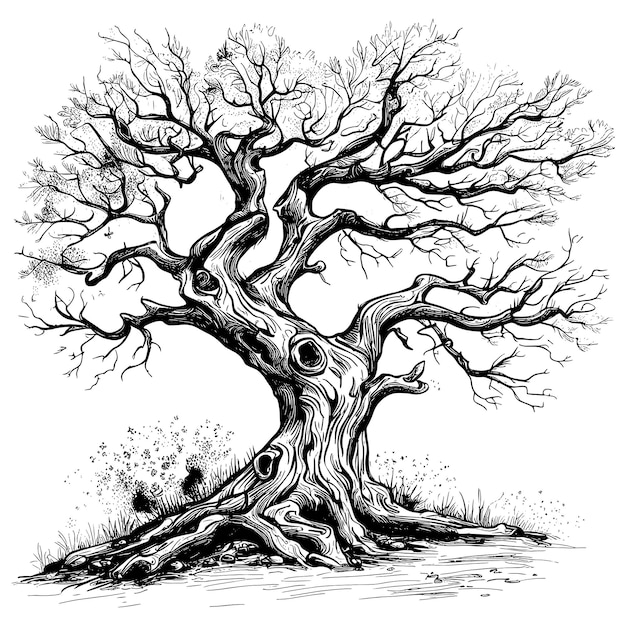In this black and white artistic depiction, the image features an extremely old, gnarled tree with a thick trunk and wide, extensive root system that appears to be partially exposed above the ground. The tree reaches upward with numerous barren branches that continually subdivide, creating a dense network of twigs without leaves. Notable features include multiple large knots and holes in the trunk, suggesting age and perhaps use by animals as nests. At the base of the tree, thin grass and a few rocks are scattered. The background is entirely white, giving the image a stark, minimalist appearance and emphasizing the intricate details of the tree itself. The image, presented in a vertically rectangular (portrait) orientation, has no visible artist signature or border.